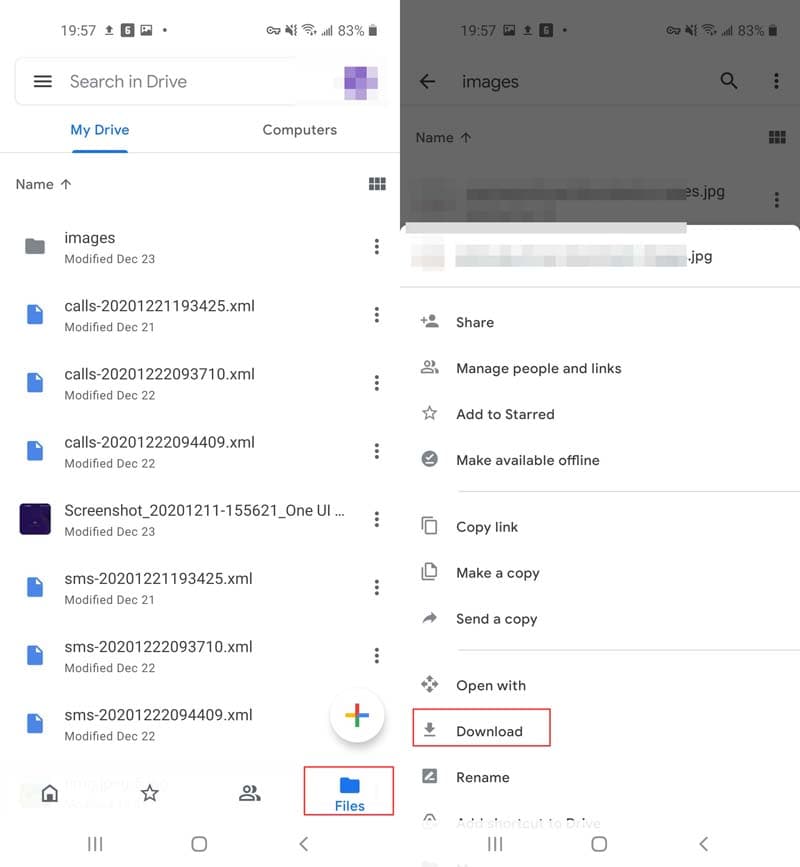The image displays a smartphone screen divided into two sections showcasing different information. On the left side, the time is shown as 19:57 with an 83% battery level. Below, a bar titled "Search and Drive" is visible, followed by two options: "My Drive" and "Computers." The "My Drive" option is selected, indicated by blue text and an underlying blue line. Beneath this, a category labeled "Name" is present, accompanied by an upward-pointing arrow.

Below, several text lines are listed. The first line reads "Images," followed by three lines starting with "cols." These lines include numerous numbers and end with ".xml." Below them is an entry labeled "Screenshot" with numerous numbers. At the bottom, three lines are titled "sms" and also end with ".xml."

At the bottom of the screen, icons for "Home," a star, a human figure, and "Files" are displayed, with the "Files" icon outlined in red. 

To the right side of the image, a pop-up menu offers several options: "Share," "Manage people and links," "Add to starred," "Make available offline," "Copy link," "Make a copy," "Send a copy," "Open with," "Download," and "Rename." The "Download" option is highlighted in red. This interface appears to be a Google Drive document page.